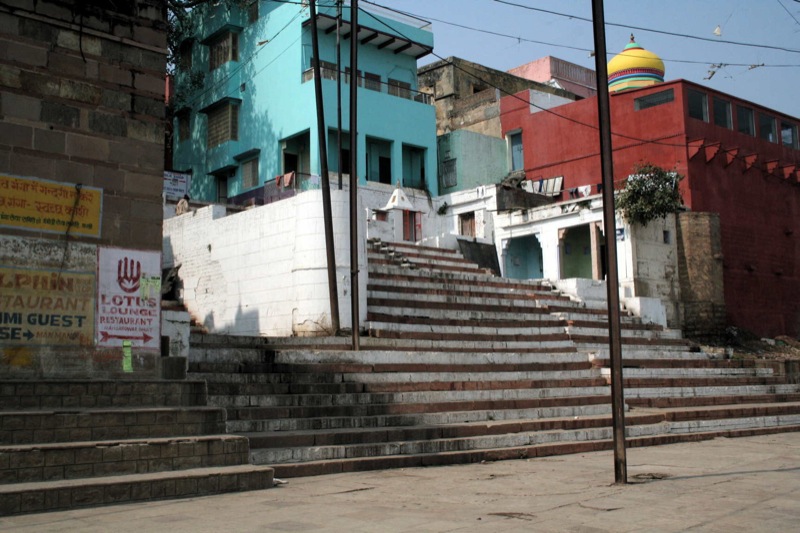The image depicts a wide rectangular photograph of an old-fashioned city block, showcasing an expansive staircase as its focal point. The staircase, slightly deteriorated, starts at the bottom left corner, ascending diagonally upwards to the right. The stairs, marked in brown and gray, lead to a multi-story, dark turquoise building centered at the top. Off to the right, the image captures a large, rusty-looking black pole extending out from the grayish-brown paved area in the foreground. To the left of the staircase, there's a brick-tall object adorned with various business advertisements, including a sign for "Lotus Lounge Restaurant" and a red arrow pointing right. The cityscape in the backdrop consists of numerous square buildings, with a prominent one in the center—painted light blue and featuring balconies and windows. To the right of the blue structure stands a red building with white accents on the first floor and a striking yellow dome on top, adorned with green and red stripes. The overall aesthetic exudes an old city charm, amplified by the aged steps and eclectic architecture.